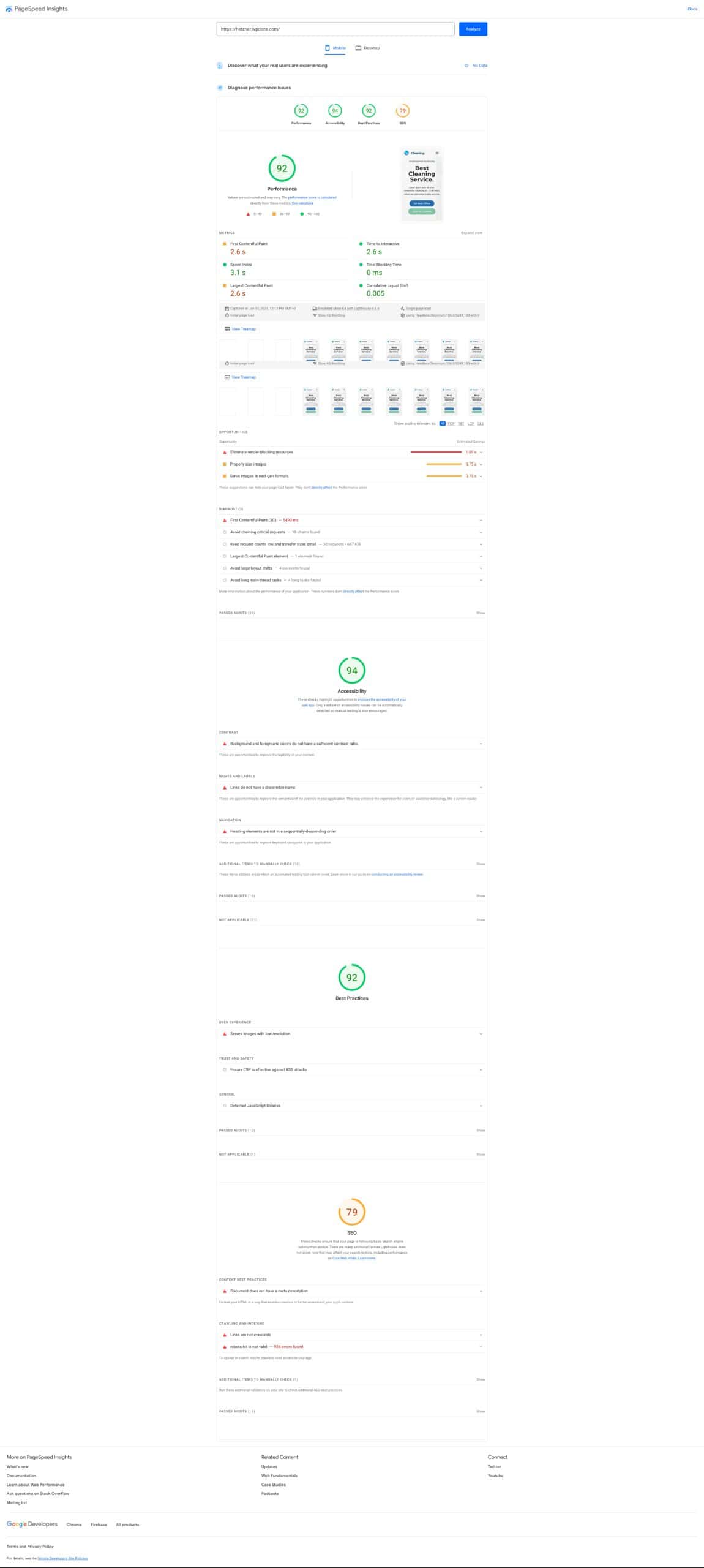In this zoomed-out image, the intricate details are somewhat blurred, yet numerous elements are discernible. At the top of the image, there's a text box containing black writing, adjacent to a blue rectangular button. Below this, green and black text is visible. Further down, three green-outlined circles with black writing underneath are noticeable, alongside a red circle with black writing below it.

Descending the layout, a green circle with black writing inside and beneath it comes into view. Neighboring this, various black and gray text elements are arranged. A blue rectangle overlays a green rectangle in this section, followed by several smaller rectangles, each topped with a brown segment and appearing green underneath.

Three distinct lines intersect the scene: a long red line, a shorter yellow line, and an orange line. Continuing downward, another green circle with black writing inside and beneath it is present, closely followed by yet another green circle featuring similar writing.

At the very bottom, an orange circle is depicted, rounding out the detailed yet distant depiction captured in this image.